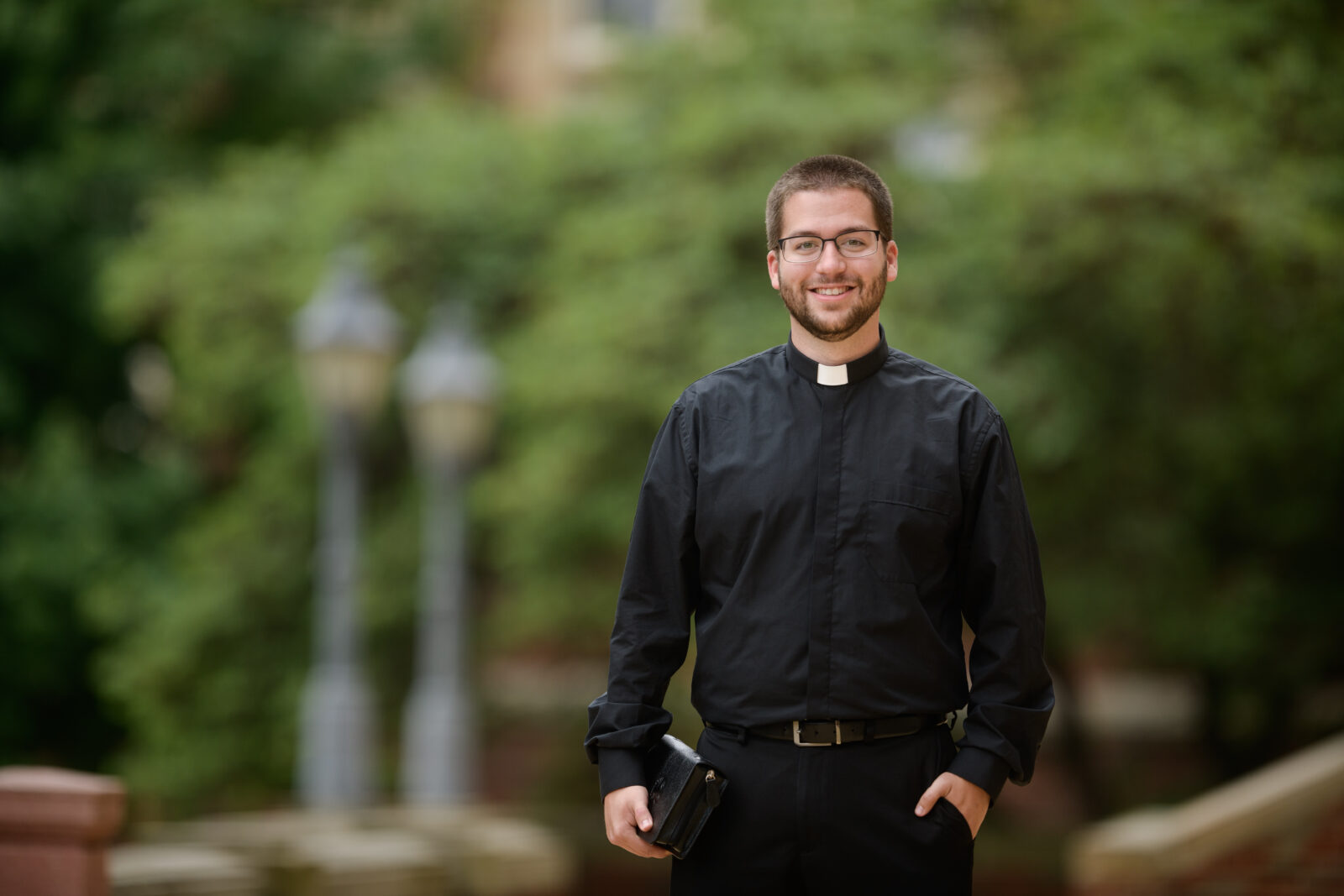The photograph captures a man, likely a priest, from the waist up. He's dressed in a long-sleeved button-up black shirt with a rigid collar overlaid by a white clerical collar, paired with black pants and a black leather belt featuring a silver square belt buckle. His left hand is partially in his pocket, thumb hooking the front, while his right hand firmly clasps a black book, presumably a Bible. Black-rimmed glasses frame his face, complementing his brown hair, beard, and mustache. The background, though blurred, reveals a daytime park setting with green trees, multiple pedestrian walkways, and silver street lamps. Additional background details include a pillar and part of a wall made of brick and lighter stone, along with glimpses of a building and its windows.